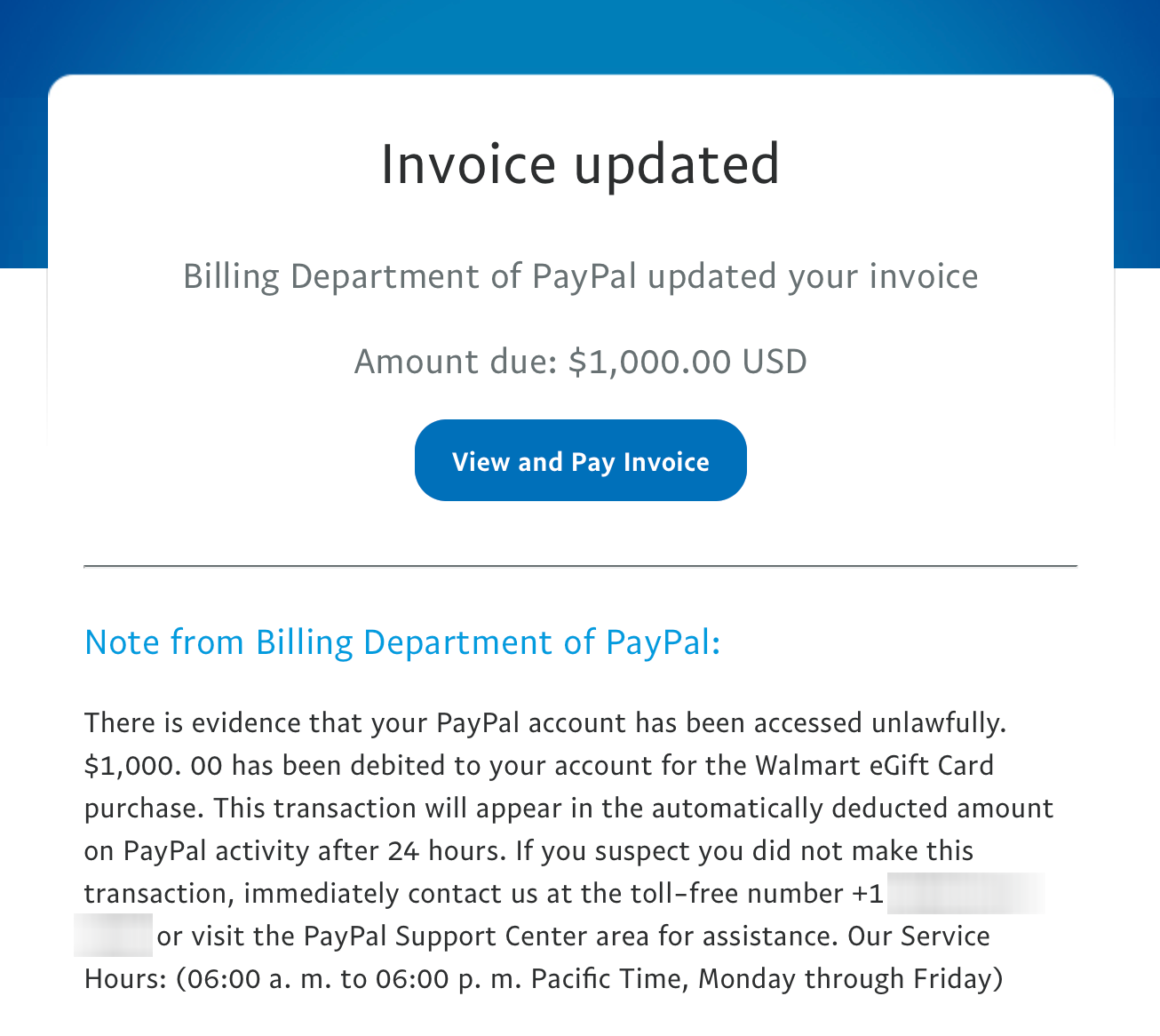This detailed caption describes a screenshot of a suspicious website purportedly from PayPal.

---

The image captures a screenshot of a website, presenting itself as a notification from PayPal. At the top of the screenshot is a blue banner, setting off the section below it. The background beneath this banner is white.

Starting from the top, in bold black text, the message reads: "Invoice Updated". Directly below, in gray text, it states: "Billing Department of PayPal updated your invoice amount due: 1,000 USD". Below this notification, there is a prominent blue action button labeled "View and Pay Invoice".

Separating this section from the content below, a horizontal gray line is evident. Under this divider, there is blue text that states: "Note from Billing Department of PayPal". 

The note elaborates that there is evidence suggesting the user's PayPal account has been accessed unlawfully, leading to a charge of $1,000 for the purchase of a Walmart e-gift card. It further explains that this transaction will appear as an automatically deducted amount in the user's PayPal activity after 24 hours.

Alarmingly, it advises that if the user suspects they did not make this transaction, they should immediately contact the provided toll-free number. The layout and urgency of the message suggest that it could be an attempt to deceive the user into responding.